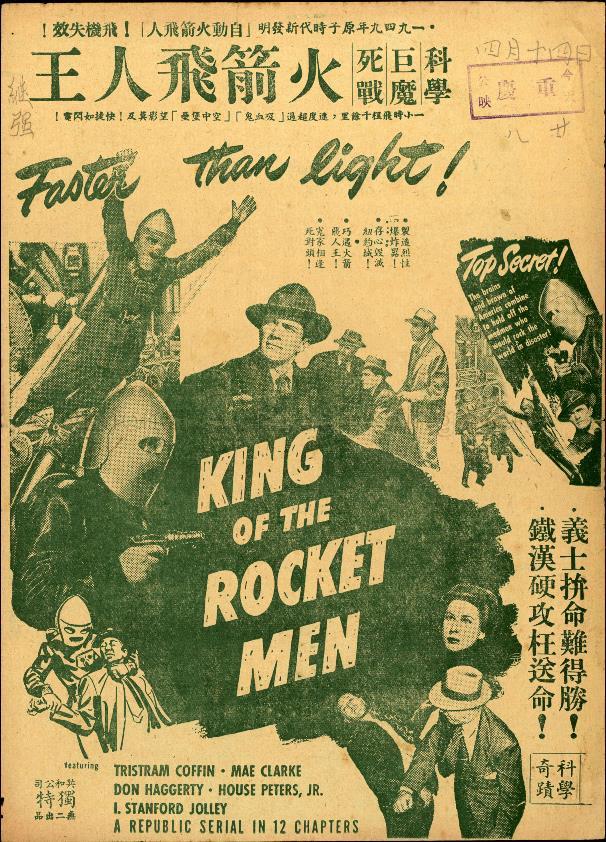This image appears to be a vintage magazine cover or a page from an old magazine, styled like a movie poster and featuring dual-language text in English and traditional Chinese. The overall background is a worn, peach-colored or light brown hue, giving it an aged appearance. Centered prominently is the title "King of the Rocket Men," accompanied by phrases like "Faster than Light" and "A Republic Serial in 12 Chapters." These descriptions suggest a serialized mystery or action-adventure theme. 

The visual elements are rendered in black and white, highlighting various figures in dramatic poses. One man, possibly the protagonist, stands out with his arms raised and a jet pack strapped to his back. Another man solemnly faces the viewer, adding a serious tone. Additionally, scenes depict men in old uniforms and hats, some engaged in combat—two men are seen fighting, and another man in a mask is shown overpowering an opponent, hinting at the action-packed nature of the series.

The layout includes traditional Chinese characters in dark green, presumably providing translations or additional context about the movie. Among the text, phrases like "top secret" and "Kristen Coffin" (though this part is unclear) are interspersed, enhancing the mysterious aura of the cover. The combination of worn paper texture, dramatic black and white visuals, and bilingual text all contribute to an evocative representation of a mid-20th-century serialized movie cover.